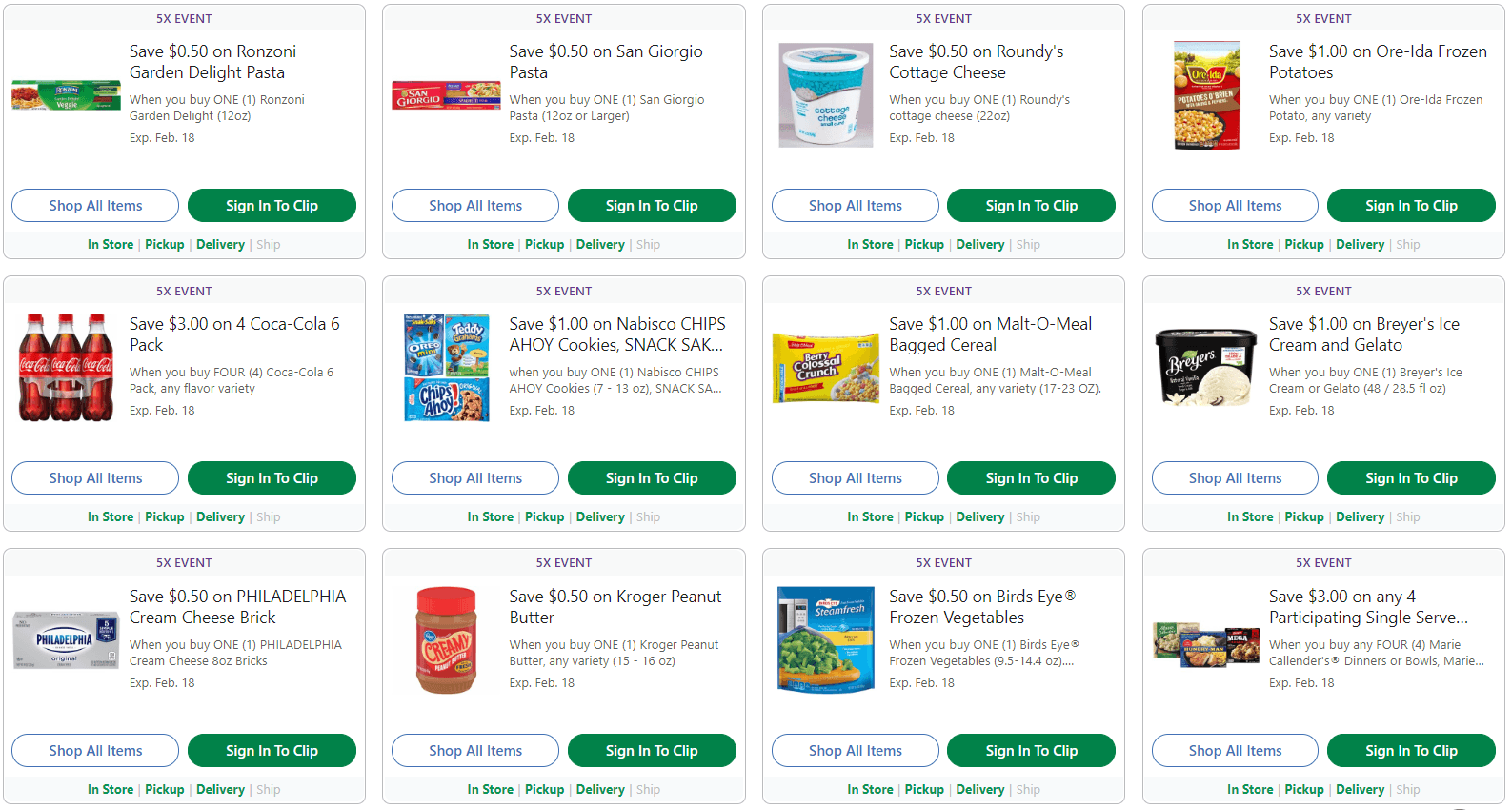Screenshot of a promotional flyer with a white background featuring various food items and corresponding coupon discounts. The coupons offer the following savings:

- Save 50 cents on Manzoni Garden Delight Pasta.
- Save 50 cents on San Glorio Pasta.
- Save 50 cents on Roundies Cottage Cheese.
- Save one dollar on Burrata Frozen Potatoes.
- Save three dollars on Four Cola Dash Cola (6-pack) or Coca-Cola (6-pack).
- Save one dollar on Nabisco Chips Ahoy Cookies.
- Save one dollar on a Cream Cheese Snack Pack.
- Save one dollar on Malt-O-Meal Bag Cereal.
- Save one dollar on Breyers Ice Cream and Gelato.
- Save 50 cents on Philadelphia Cream Cheese.

The text "CHIPS AHOY" and "SNACK" are capitalized, with "SNACK" followed by an ellipsis. The Philadelphia Cream Cheese text is in all caps as "PHILADELPHIA".